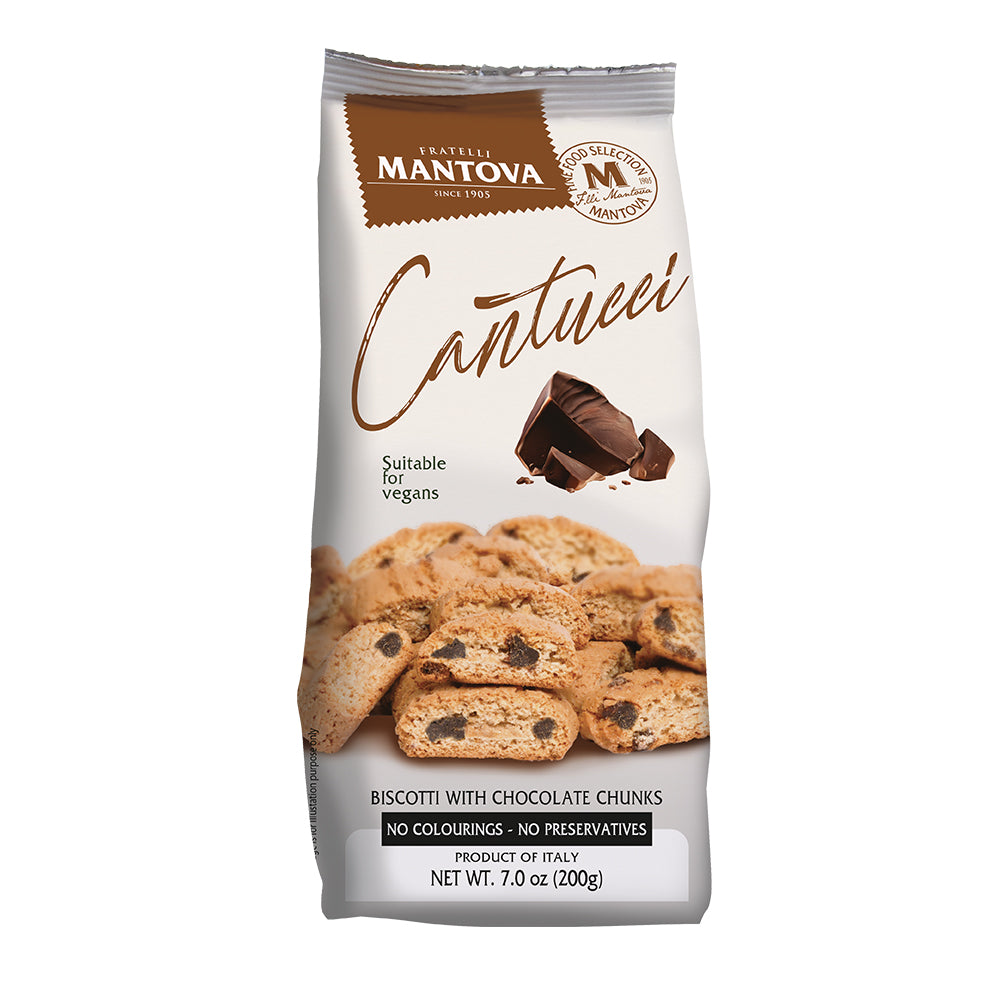This is a centered photograph of a white paper bag containing biscotti with chocolate chunks, produced by Fratelli Mantova since 1905. The brand name "Cantucci" is prominently displayed in fancy brown cursive letters, alongside claims of being suitable for vegans and free from colorings and preservatives. The packaging features a brown and white diagonal square logo at the top left corner, which reads "FRATELLI MANTOVA" in white text, along with a seal indicating the product's fine food selection. Pictured prominently on the front of the bag is a pile of biscotti, some broken to reveal chocolate chunks inside, with a crumbled chocolate bar floating above them. Additional details include the product weight of 7.0 ounces (200 grams), and a small text banner stating "No colorings, no preservatives" beneath the image of the cookies. Note that the image of the cookies is marked for illustration purposes only.